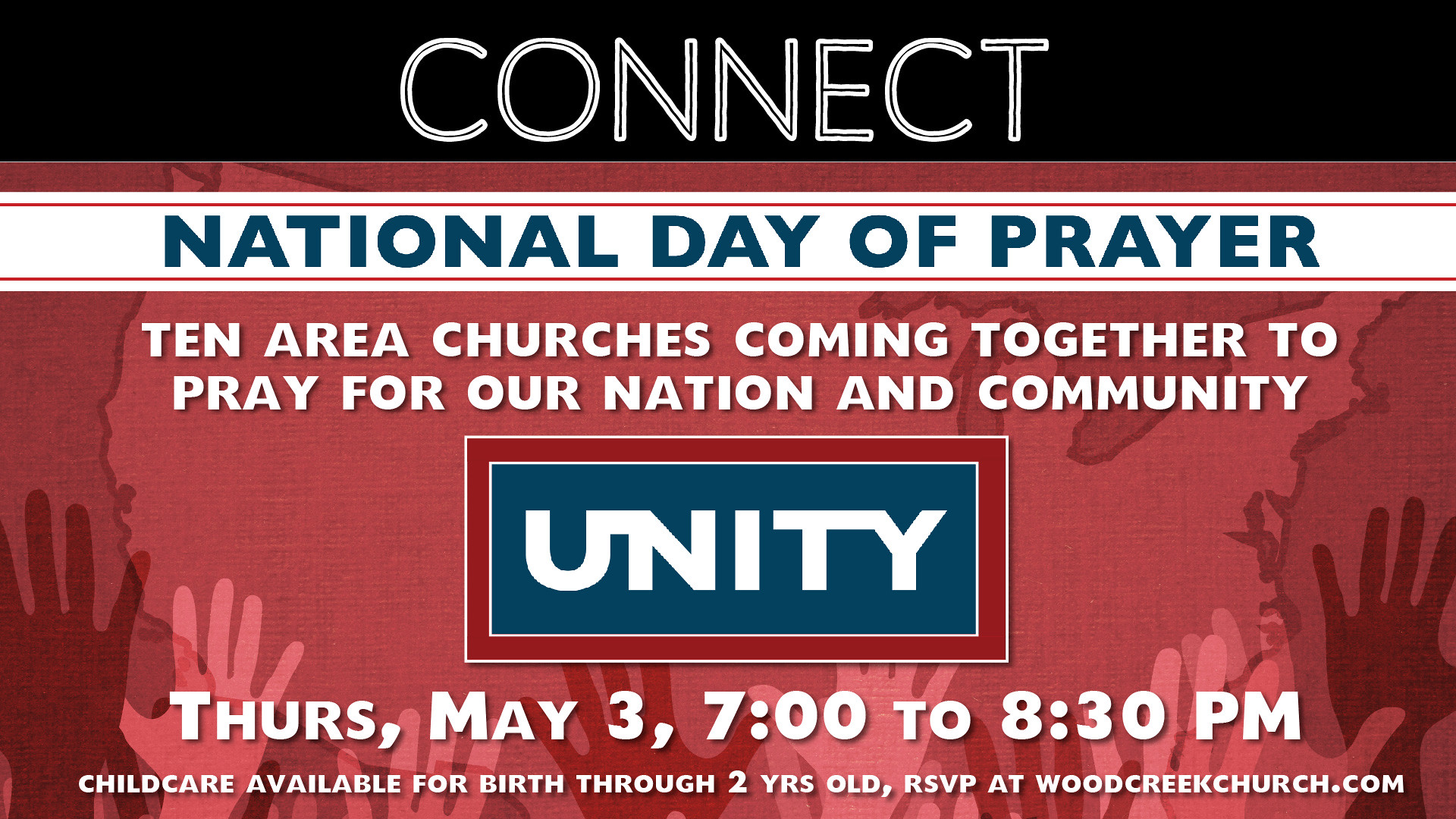This advertisement for a church event features a prominent "Connect" label at the top in white text on a black bar. Below it, a maroon bar is followed by a white band with bold blue text announcing the "National Day of Prayer." The main section has a vivid red and purple background, showcasing the outline of the United States alongside silhouettes of hands in prayer. Bold, white text proclaims, "10 Area Churches coming together to pray for our nation and community." A blue box lower in the design highlights the word "Unity" in white text. At the bottom, detailed event information includes "Thursday, May 3rd, 7:00 to 8:30 PM," and notes that childcare is available for children from birth through 2 years old. Attendees are invited to RSVP at woodcreekchurch.com.